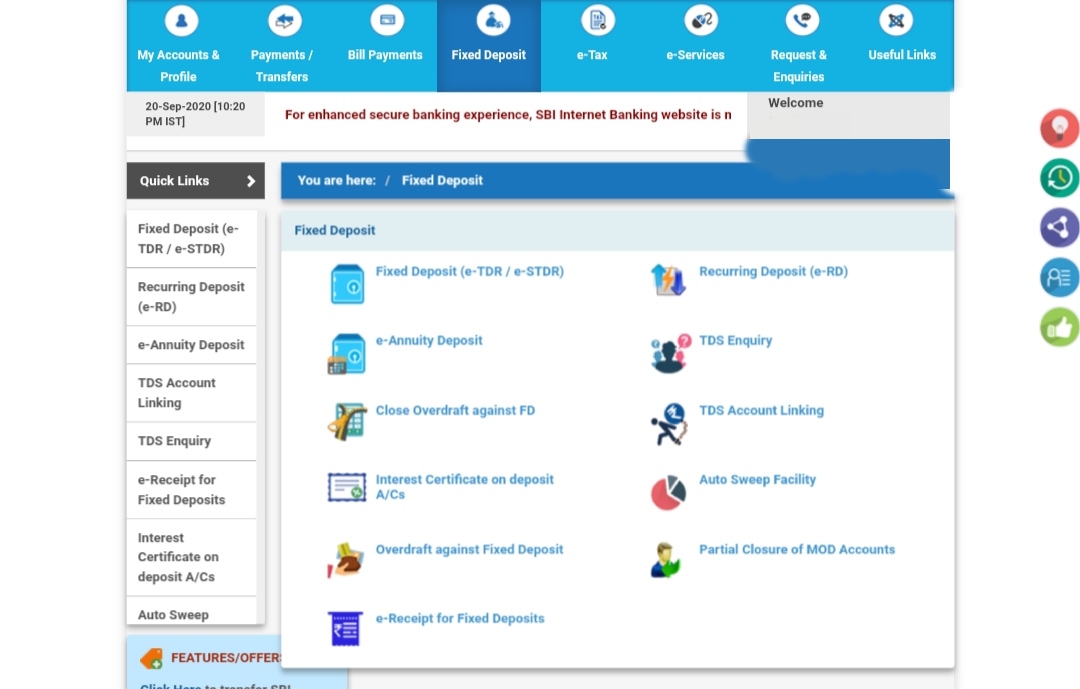The website features a structured layout for enhanced navigation and banking services. At the top, a header presents multiple selections arranged horizontally from left to right: "My Accounts and Profile," "Payments/Transfers," "Bill Payments," "Fixed Deposit," "e-Tax," "e-Services," "Requests and Inquiries," and "Useful Links." Each item is paired with a circular logo above it, set against a blue background with white text.

Below the header, a horizontal section displays the date "20 September 2020" accompanied by a message in red text, "For enhanced secure banking experience." However, the message cuts off unexpectedly, followed by a "Welcome" note.

As we proceed further down, another line in blue and white text indicates the user's current location within the site: "You are here, Fixed Deposit." On the left side, a vertical menu titled "Quick Links" offers several options including: "Fixed Deposit," "Recurring Deposit," "e-Annuity Deposit," "TDS Account Linking," "TDS Inquiry," "e-Receipt for Fixed Deposits," "Interest Certificate on Deposit Accounts," and "Auto Sweep."

The middle section features a comprehensive list related to fixed deposits, organized into two columns:
- Fixed Deposit
- e-Annuity Deposit
- Close Overdraft Against FD (Fixed Deposit)
- Interest Certificate on Deposit Accounts (ACs)
- Overdraft Against Fixed Deposit
- e-Receipt for Fixed Deposits
- Recurring Deposit
- TDS Inquiry
- TDS Account Linking
- Auto Sweep Facility
- Partial Closure of MOD Accounts

To the far right of the webpage, five icons are vertically stacked outside of the main content area. The overall design emphasizes ease of access and security for users navigating their banking needs.